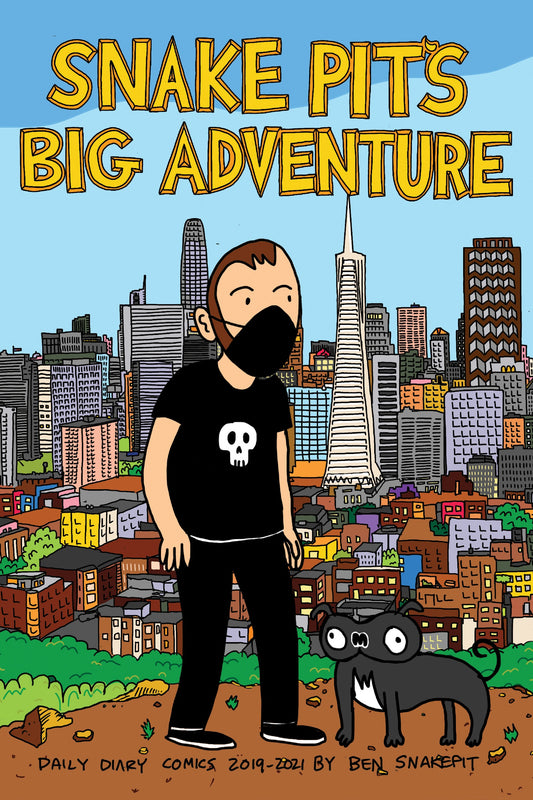A vibrant comic book cover features a sprawling, bustling cityscape under a vast blue sky that gradually lightens towards the horizon. Prominent skyscrapers reach for the heavens, while rows of apartment buildings stretch towards the viewer, creating a sense of depth and urban density. Dominating the center is a striking white building crowned with an antenna or steeple, standing as a focal point in the sea of architecture. In the foreground, a gentleman clad in a black short-sleeved t-shirt emblazoned with a white skull pairs his ensemble with matching black pants. A sleek black mask conceals his face, adding an air of mystery. At his side, a whimsically cartoonish dark grey dog, characterized by patches of white on its chest and bulging white eyes, stands out, adding a touch of humor and charm to the otherwise dramatic scene.